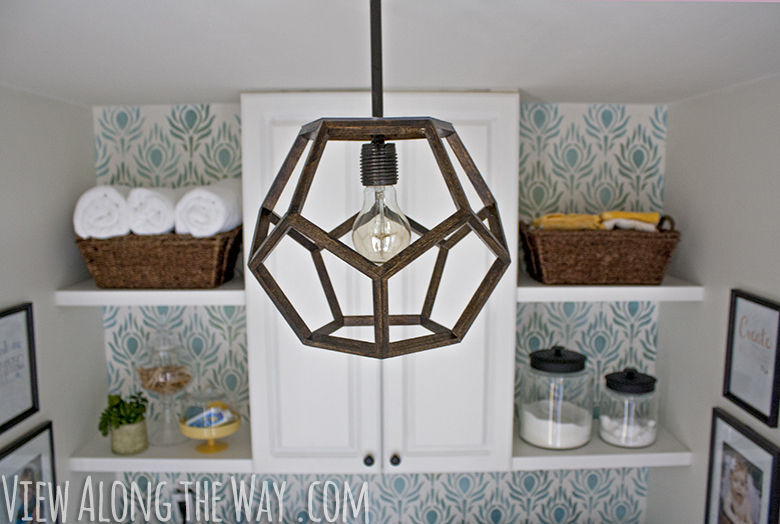This image captures a charming kitchen scene, with the focal point being a unique wooden chandelier designed in a geometric, possibly dodecahedron-shaped frame. The light fixture hangs from a slender, straight pole extending from a black cylinder mounted on the ceiling. Encased within the wooden framework is a light bulb that casts a warm glow in the small, cozy room. The backdrop features white cabinets flanked by two white shelves on either side. The left shelf holds neatly folded towels and decorative vases, while the right displays glass jars filled with flour and sugar. Both shelves are adorned with tasteful baskets. The wallpaper behind the shelves showcases a delicate blue floral pattern, complementing the white-painted walls. Framed art, including images of children and food recipes, adds a personal touch to the space. The bottom left corner of the image contains the text "viewalongtheway.com" in white. Overall, the detailed and tidy arrangement highlights the inviting and well-organized nature of this kitchen.